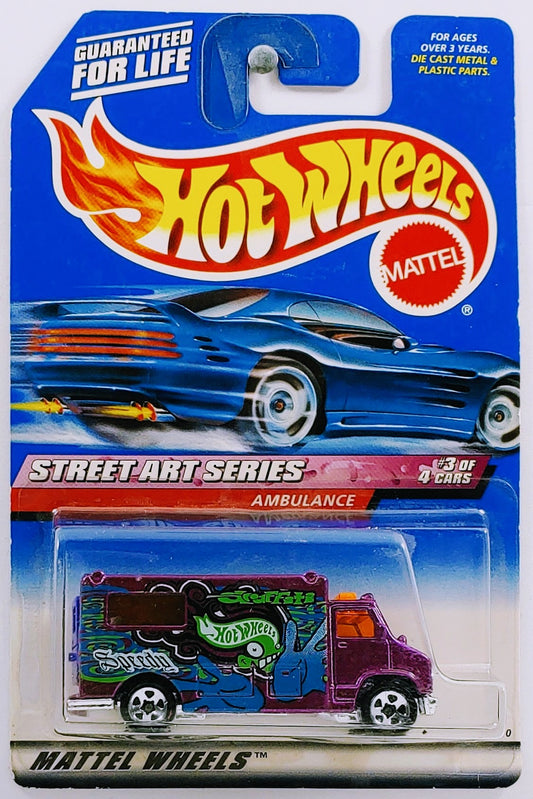The image features an unopened Hot Wheels toy package in pristine condition. The packaging prominently showcases the iconic Hot Wheels logo, featuring yellow "Hot Wheels" lettering on a flaming red banner, with the word "Mattel" encased within a circle at the base of the flame, signifying the brand. Above the logo, "Guaranteed for Life" is stamped in white text on one of the flame tips.

In the top right-hand corner of the package, it states, "For ages over three years," indicating the toy's safety for young children. Adjacent to this is another note that reads "Die-cast metal and plastic parts" in yellow text, emphasizing the construction materials used.

The packaging background is predominantly blue, giving the whole presentation a cool, vibrant feel. Below the main logo, there's a dynamic image of a blue car, possibly a Camaro, depicted as if it's speeding away, with a trail of white tire smoke illustrating movement. This sets the stage for the "Street Art Series" label in red background with white letters, identifying this toy as part of a unique collection. It also notes this is the third car in a series of four.

The main attraction, a toy ambulance, is sealed in clear plastic within the package. However, this isn't a standard ambulance; it boasts a subtle purple wine color with green graffiti-style text spelling out "Speedy" alongside blue hands forming a peace sign. The lower part of the package identifies the series and brand with "Mattel Wheels™" written in black and white.

Overall, the detailed and vividly illustrated packaging conveys a sense of excitement and collectibility, appealing to both young enthusiasts and adult collectors.